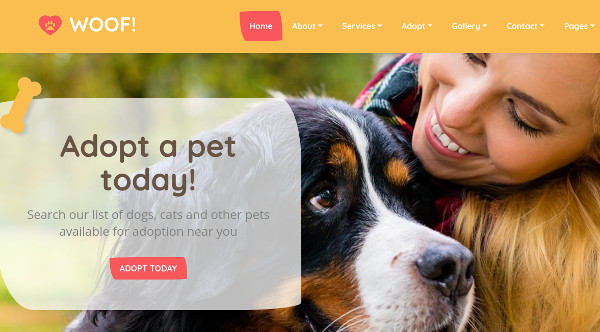The webpage for WOOF! features a clean, modern design with the company name prominently displayed in all caps, in a white sans-serif font. Next to the name is a pale red heart with an orange paw print superimposed on it. At the top of the page, a full horizontal banner in pale orange serves as a background for the navigation links.

The navigation bar includes links for "Home," "About," "Services," "Adopt," "Gallery," "Contact," and "Pages," each accompanied by a dropdown arrow. The "Home" tab is highlighted with white text on a pale red, irregularly shaped trapezoid.

The background image of the website features a blurred depiction of trees with a partial view of a Bernese Mountain Dog's head. Beside the dog is a female face, partially visible, with one eye fully shown and a partial view of the other. She has a wide smile, dimples, and blonde hair cascading over her shoulder.

Superimposed on the Bernese Mountain Dog is a pop-up message that reads "Adopt a Pet Today," styled similarly to the "Home" button on a pale red trapezoid. Below this message, there is text encouraging visitors to search for adoptable dogs, cats, and other pets nearby. At the bottom of the pop-up, a longer trapezoid in the same style contains the call-to-action "Adopt Today" in all caps and white font. 

In the top left corner of the pop-up is an orange bone icon, adding a playful touch to the design.